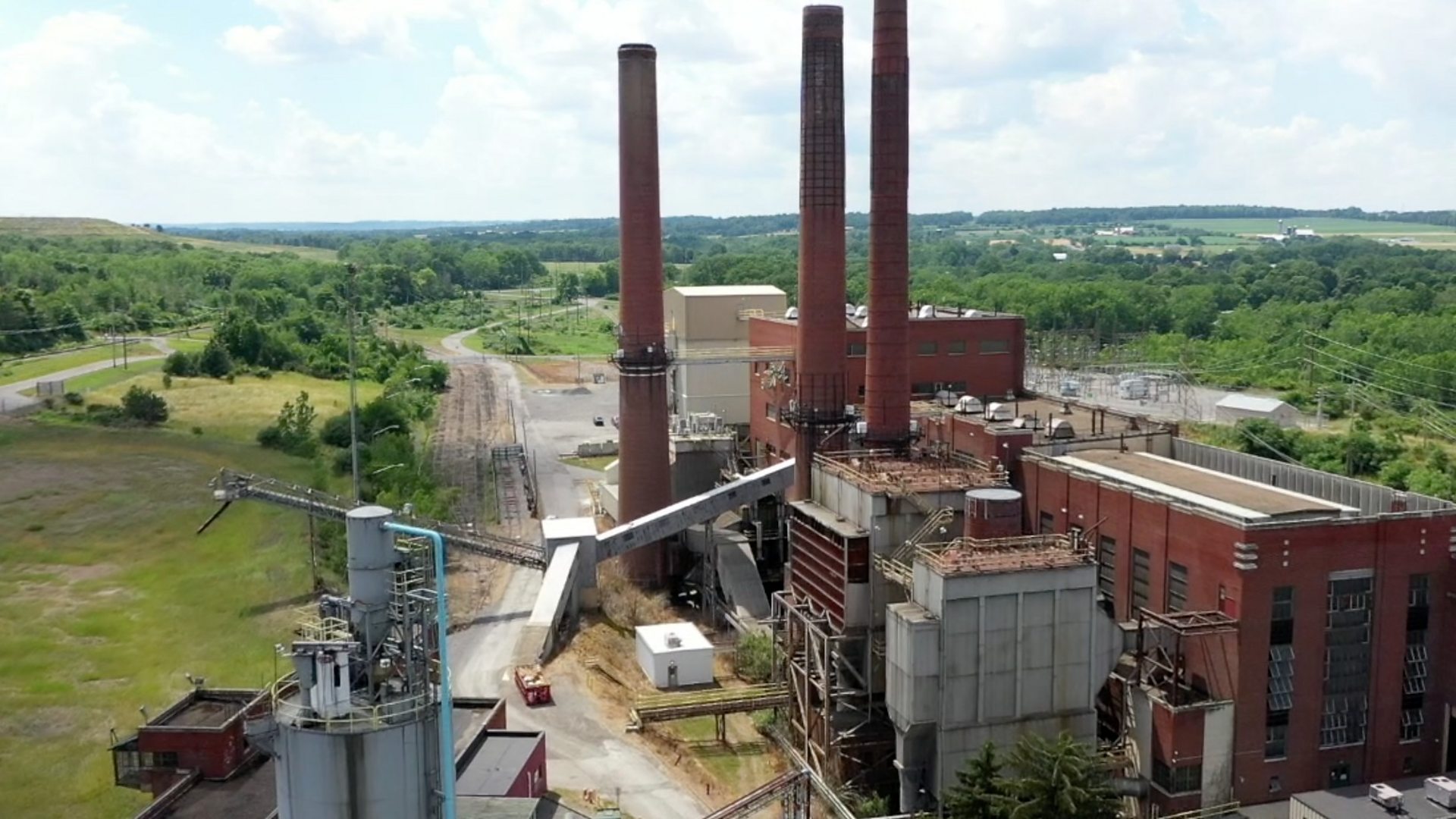The photo captures a wide, panoramic view of an industrial building, primarily composed of red brick. Dominating the center-right of the image, the structure features three tall, cylindrical smokestacks and several smaller gray structures, including towers and box-like units. The building is surrounded by a plethora of industrial elements such as conveyor belts and tubes that weave through the facility. On the left side of the building, a hard dirt or gravel road runs parallel, extending into the distance and flanked by lush green trees and countryside, indicating a remote, rural setting. In the far distance, the landscape is dotted with a few buildings, all under a sky filled with white, fluffy clouds. The scene has a bucolic charm despite the industrial presence, with an overall sense of being immersed in a serene, yet functional, rural environment.